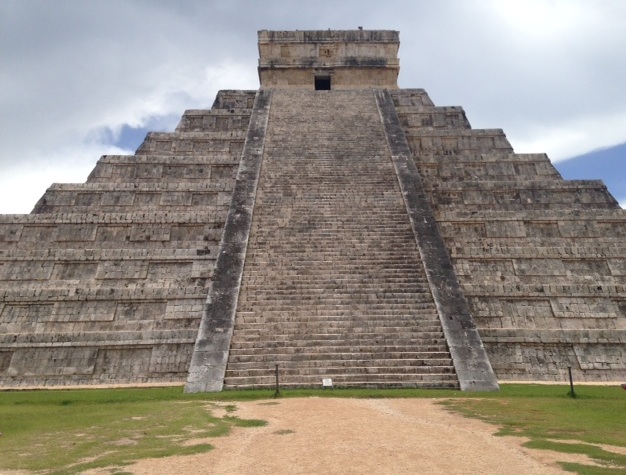The image depicts a large, stone-tiered pyramid, possibly an Aztec structure located in Mexico. The pyramid features a wide set of stairs that ascend from the base to a rectangular structure at the top with an open doorway. The pyramid itself is made entirely of stone and is terraced with multiple levels leading up to the top. In front of the pyramid, there is a dirt pathway flanked by green grass, with additional patches of grass at the base of the structure. The scene is set under a mostly cloudy sky, with some blue peeking through, and it is daylight, casting a bright light over the landscape. There are poles, possibly forming a gate, near the base and what looks like a white sign at the bottom of the staircase. The atmosphere combines natural elements with the historic grandeur of the pyramid.